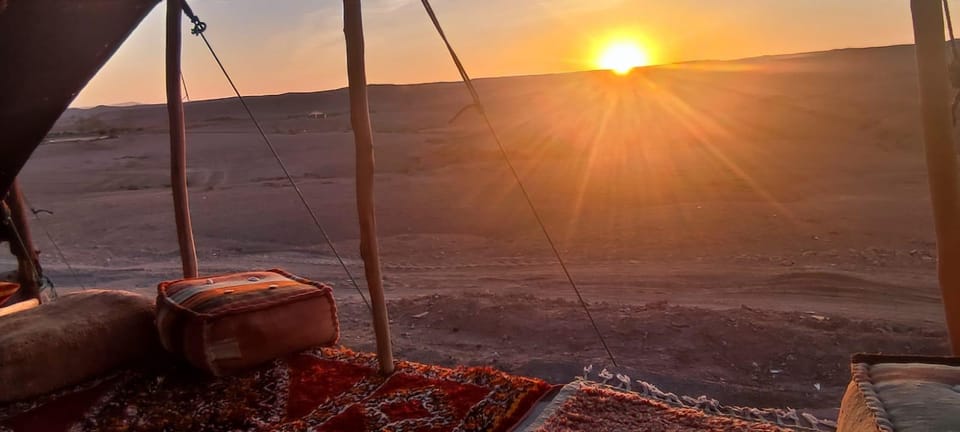This photograph captures a serene desert sunrise, with the sun peeking over the horizon formed by a large sand dune. The sky is bathed in a warm palette of oranges and yellows, accentuated by a subtle lens flare. The image is taken from the interior of a tent, as indicated by several visible wooden poles supporting the canvas structure. The front of the tent is open, providing an unobstructed view of the breathtaking landscape. The floor of the tent is adorned with Persian rugs featuring intricate white and black designs that stand out against a red background, while large throw pillows are arranged for seating. Scattered rocks are visible on the ground outside, adding a touch of rugged authenticity to the scene. Overall, this image evokes a peaceful and immersive desert experience, potentially set in the Middle East or the Sahara Desert.